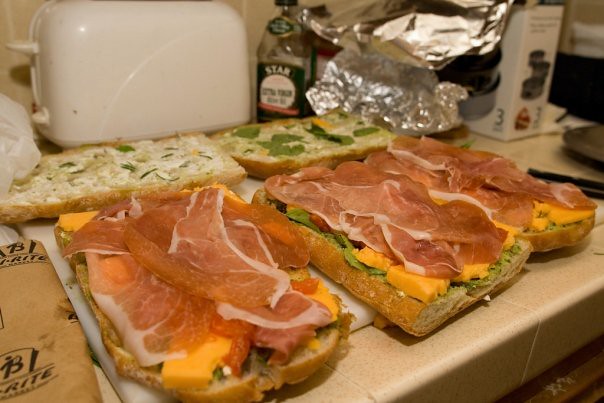The image depicts a detailed sandwich-making scene on a white cutting board placed atop a beige tile counter. Centered in the frame are three open-faced Italian-style sandwiches made from wide, crunchy ciabatta bread. The sandwiches are generously layered with thinly sliced prosciutto, chunks of cheddar cheese, fresh lettuce, and possibly avocado. Around the sandwiches, additional bread pieces, likely meant to be their tops, are adorned with butter, shredded cheese, herbs, and some green leaves. In the background, a white toaster and a bottle with a green label and a white circle that says "star" can be seen. On the right-hand side, loose pieces of aluminum foil are visible next to a Reynolds wrap box, hinting at the ongoing preparation.